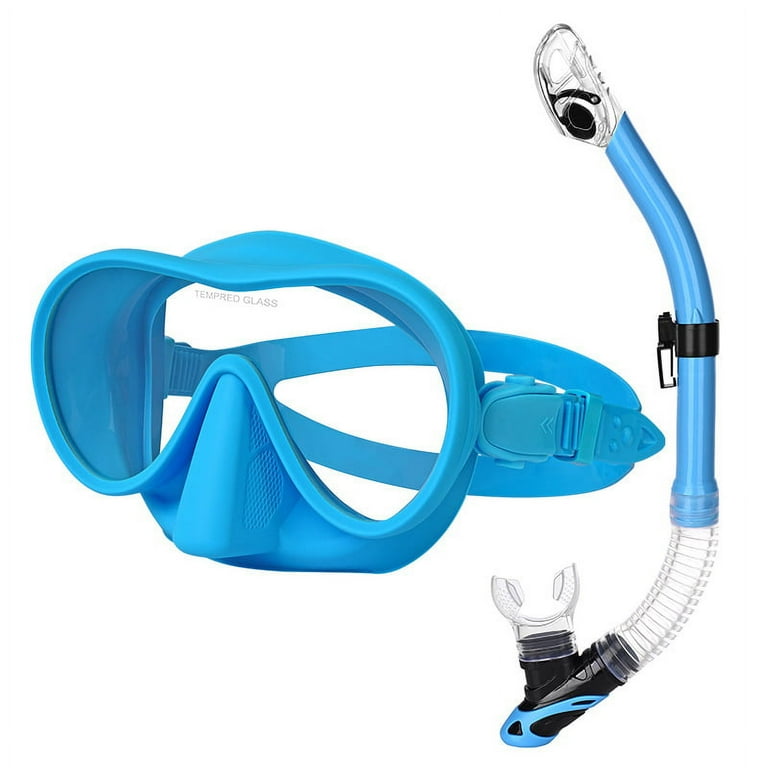This is a detailed photograph of snorkeling equipment displayed against a plain white background. At the center is a pair of blue-colored goggles with clear, anti-fog tempered glass lenses that cover both the eyes and the nose, and include an adjustable blue strap with a buckle at the back. The inscription "tempered glass" is visible on the lenses. To the right, there is a matching snorkel featuring a blue and transparent design. The snorkel starts with a clear tube that curves downward and attaches to a solid blue section which is connected by a black clasp. It continues with another transparent segment that is curved and ends in a black mouthpiece, making the overall setup ideal for underwater exploration.